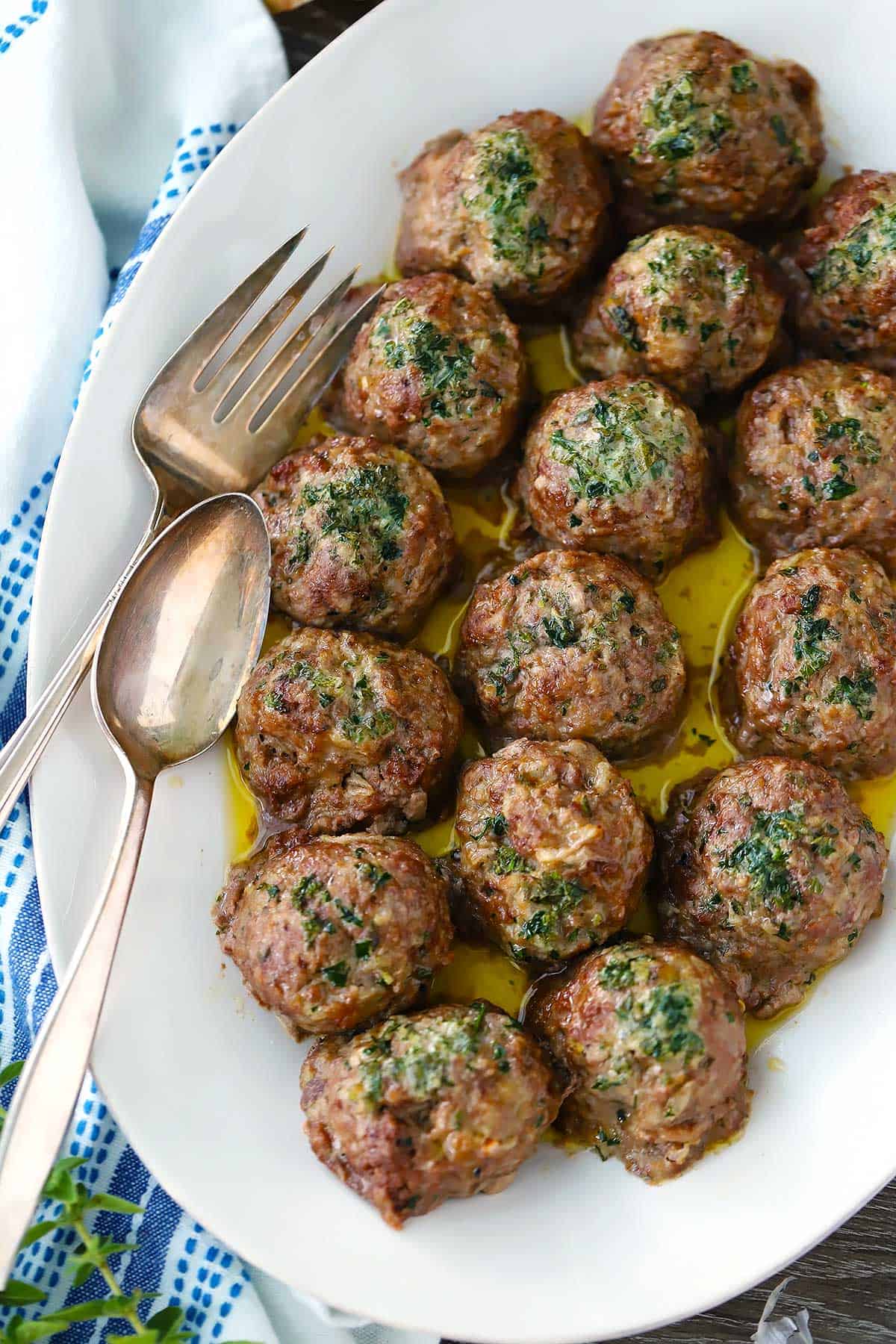This photograph showcases a beautifully arranged presentation of meatballs on a white ceramic oval serving platter, which occupies the majority of the image. The platter, slightly tilted to the right, rests on a white cloth adorned with subtle blue striping. Surrounding the pristine platter, the corners of a brown wooden table peek through at the bottom right and upper left of the composition.

The focal point of the image is the meticulously detailed meatballs, totaling between 15 to 20 in number. Each meatball is generously garnished with green herbs, likely parsley, which adds vibrant color to their charred yet appetizingly well-done exterior. The meatballs are bathed in a buttery broth or oil that glistens beneath them, heightening their appeal. 

Strategically placed on the oval platter are a clean, four-pronged copperish fork and a matching copperish spoon, both positioned to the left side, enhancing the dish's presentation. The overall staging of the photograph conveys an inviting, ready-to-serve feel, with the high-quality image focusing on the meatballs' enticing textures and aromatic seasoning.